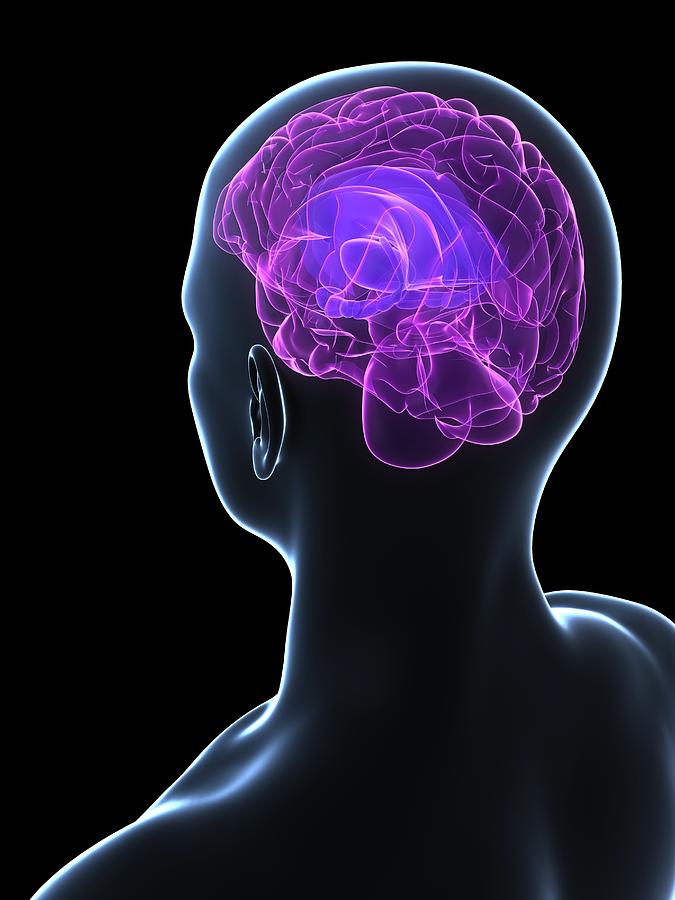The image is a computer-generated graphic featuring a human-like figure against an all-black background. The figure, resembling a mannequin or a model of a human body, stands with its back to the viewer, exposing its shoulders that extend to the left and right edges of the image. The body and outline are illuminated in a gradient of dark blue-green to light grayish tints, accentuated with glowing white lines that define the contours of the shoulders and the ear visible on the left-hand side. At the top of the image, where the brain is located, there is a mesmerizing swirl of pink and purple lights. This abstract portrayal of the brain emits fluorescent hues and intricate lines that intersect and diverge in an almost smoke-like fashion. These elements create a dynamic, almost ethereal effect, with some lines appearing to form shapes resembling hands or horns, further emphasizing the surreal and artistic nature of the depiction.